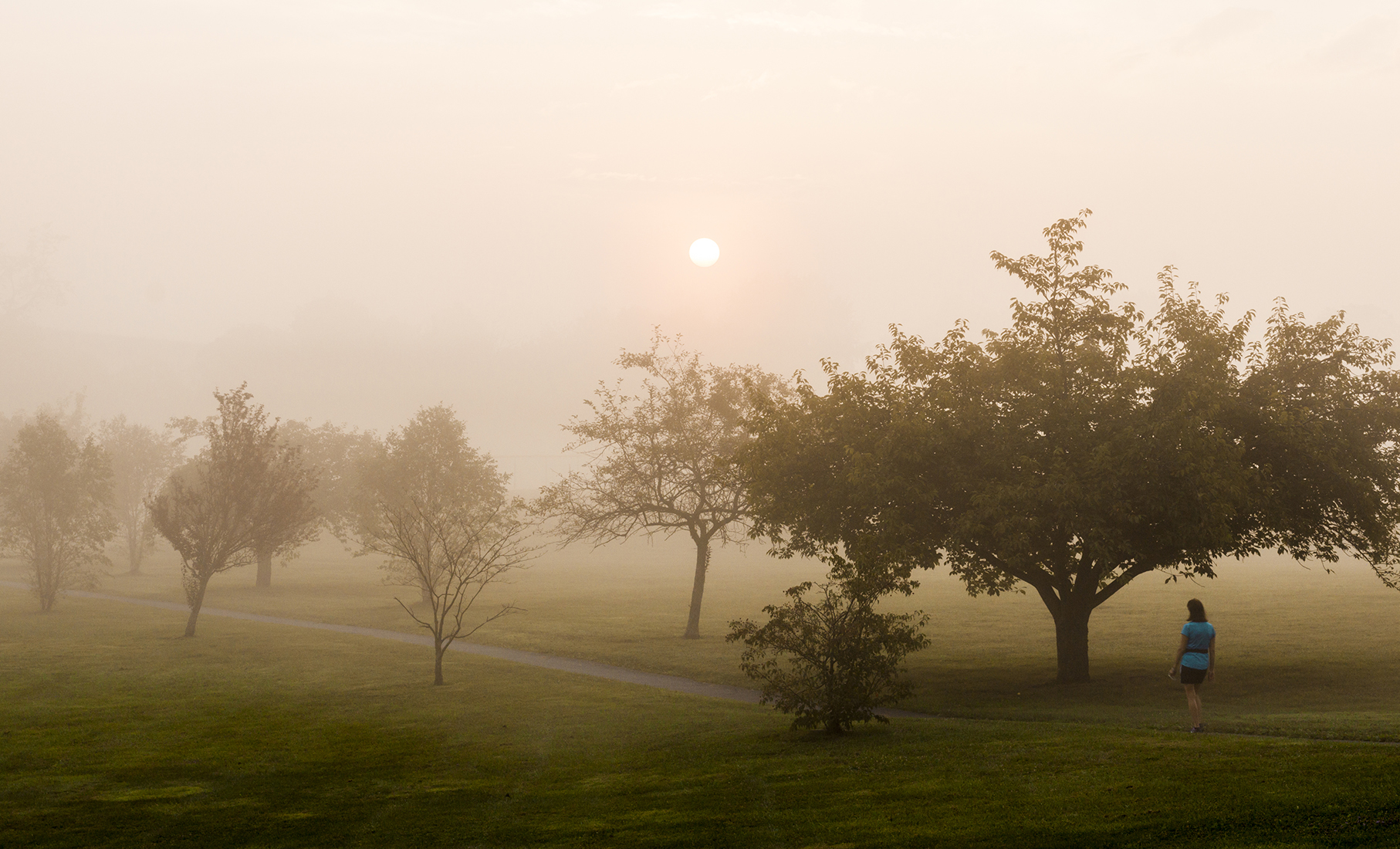In this eerie and tranquil scene from the top of a hill, an empty park stretches out before us under a foggy, yellow-tinted sky, hinting at either fog or a distant fire. The weather is hazy, with a small, white sun barely visible in the late afternoon sky. A neatly mowed, uniform green lawn lines the park, which features a man-made path starting from the bottom right and extending horizontally across the image to the lower left. Trees, uniformly spaced and seemingly planted by human hands, flank both sides of the path. The scene is sparse and quiet, with only a single woman present. Dressed in a blue t-shirt and black shorts, her long dark hair flows as she walks alone along the trail, capturing our attention as she moves from the lower right through this desolate yet meticulously maintained landscape.